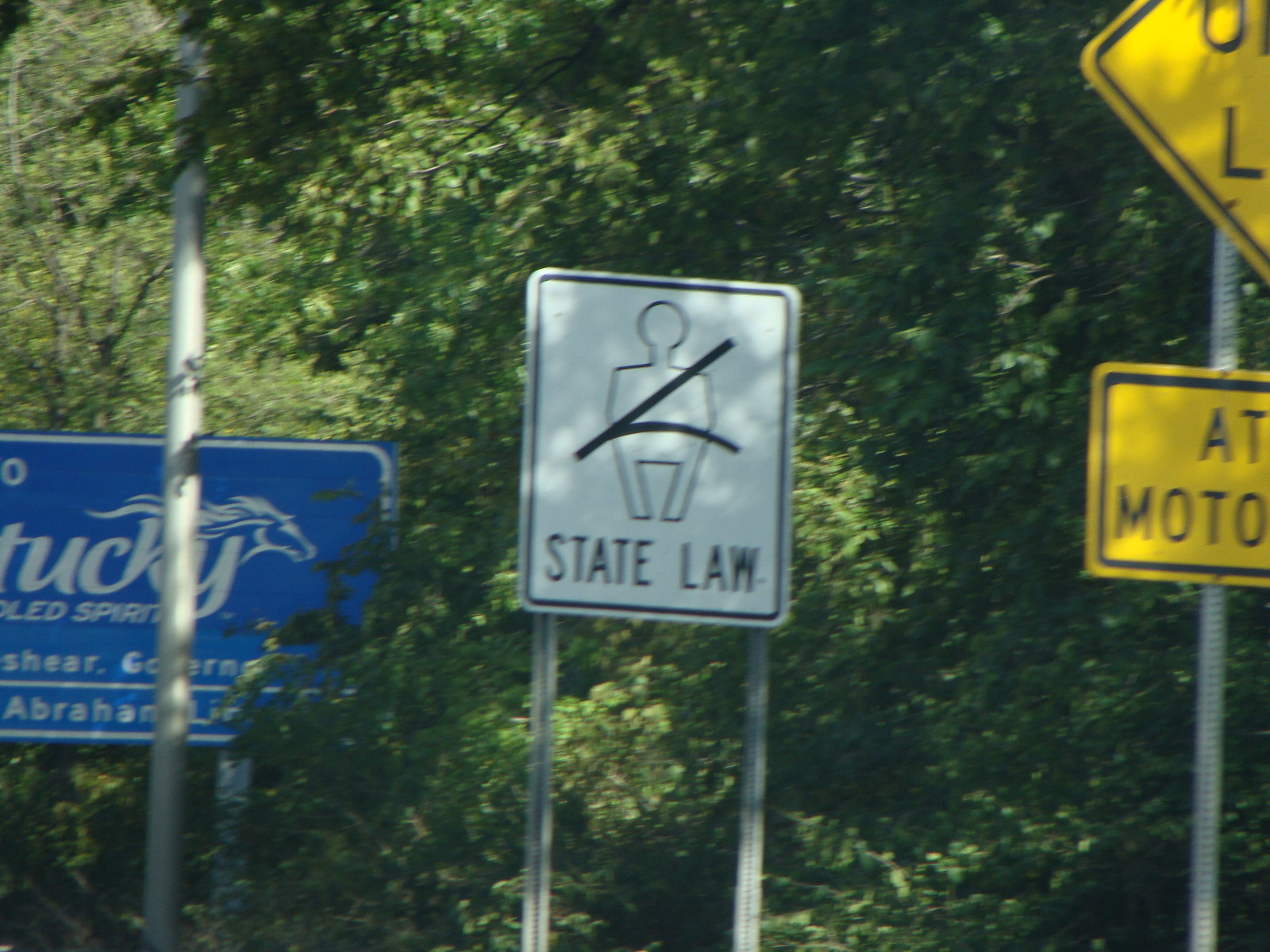The photograph appears to have been taken from a moving vehicle, indicated by its slightly zoomed-in perspective and presence of motion blur. Dominating the image is a white highway sign featuring a stick figure wearing a seatbelt, accompanied by the bold all-capitalized text "STATE LAW," emphasizing the legal requirement to wear seatbelts. In the background, lush green trees and dense foliage provide a natural backdrop. Flanking the central sign, although partially cut off, are additional roadside signs—a yellow sign to the right and a larger blue sign to the left. While the text on these signs is not legible, the blue sign distinctly features an icon of a horse. The composition and elements together paint a vivid picture of a state-regulated highway scene amidst verdant surroundings.